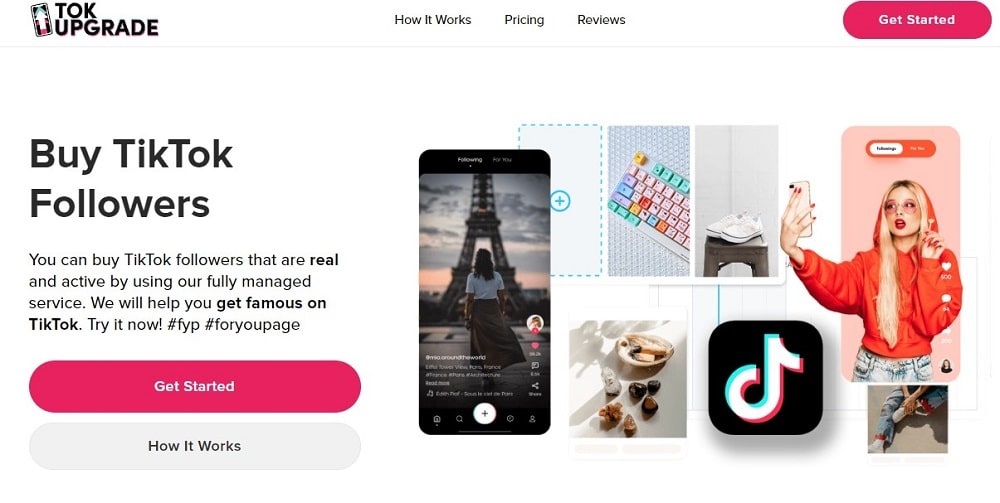[Description of the image]

The image is a promotional page for a service that allows users to purchase real and active TikTok followers. The main header reads, "Talk Upgrade: How it Works, Pricing, Reviews," followed by a prominent pink "Get Started" button. The text continues with, "Buy TikTok Followers. You can buy TikTok followers that are real and active by using our fully managed service. We will help you get famous on TikTok. Buy it now," accompanied by hashtags like "#FYP" and "#ForYouPage."

Below the main content, there's another pink "Get Started" button, followed by a section labeled "How it Works." 

A series of images are displayed underneath:
1. A girl, dressed in a white shirt and dark skirt, is facing the Eiffel Tower.
2. A colorful keyboard.
3. A seashell and rocks on a white background.
4. A pair of white sneakers on a chair.
5. The TikTok logo on a black background.
6. A girl with long blonde hair in a red sweatshirt and jeans, taking a selfie.
7. An image showing a person's legs, positioned next to each other, without further context.

The page provides a visually engaging layout to complement the promotional content and service details.